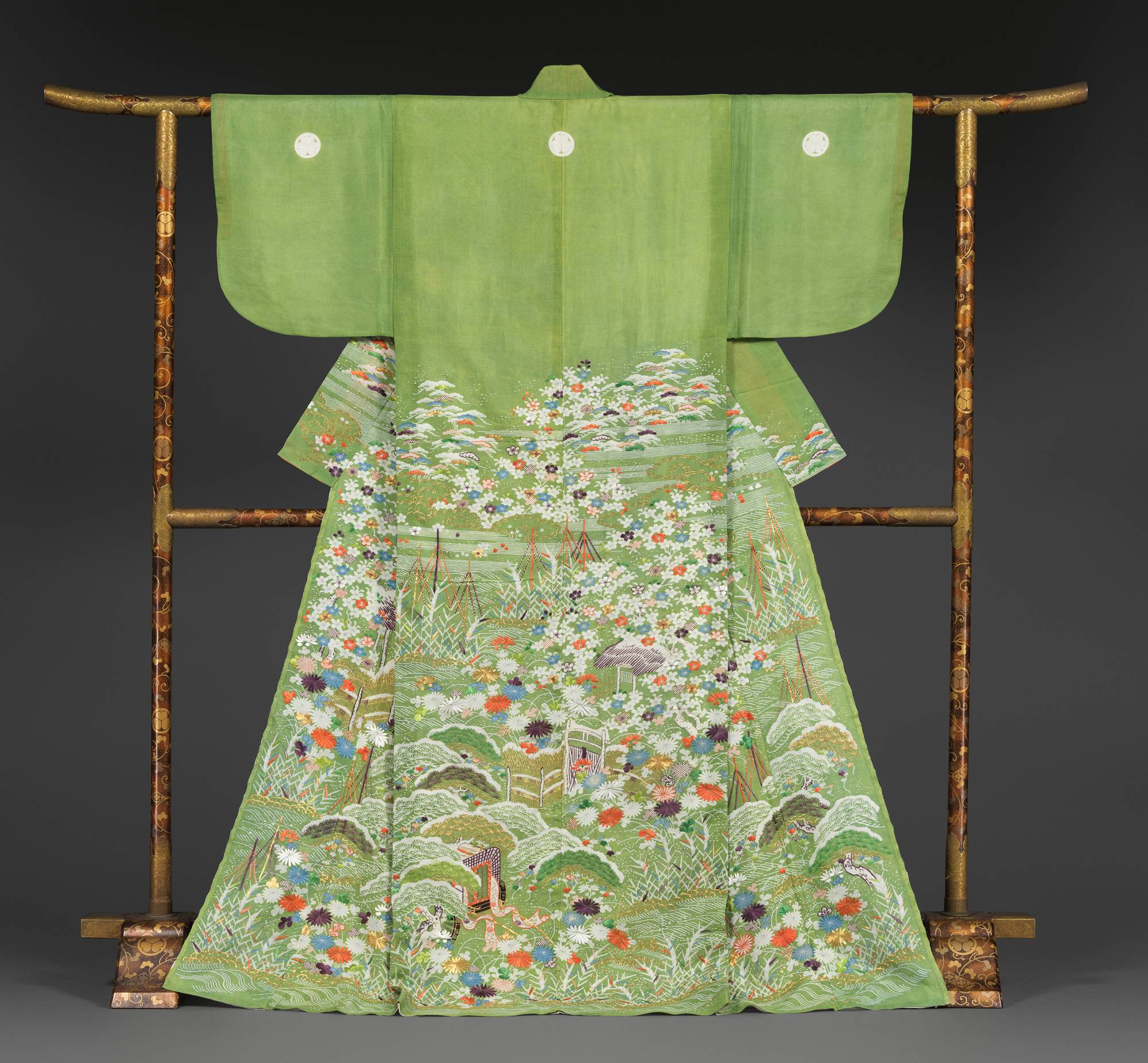The photograph captures an ornate display of a pastel green kimono, intricately adorned with elaborate floral embroidery. Set against a plain gray background, the kimono is elegantly draped over a bronze, almost gold-colored stand, which itself boasts an ornate design. The kimono's fabric resembles linen and the detailed embroidery spans from the waist down to where the knees would be if worn, featuring a vibrant array of flowers in white, orange, blue, and purple hues, evocative of a serene landscape of hills and blossoms. The meticulous display and artistic details suggest that this piece could be showcased in a museum, possibly highlighting its Asian design heritage.